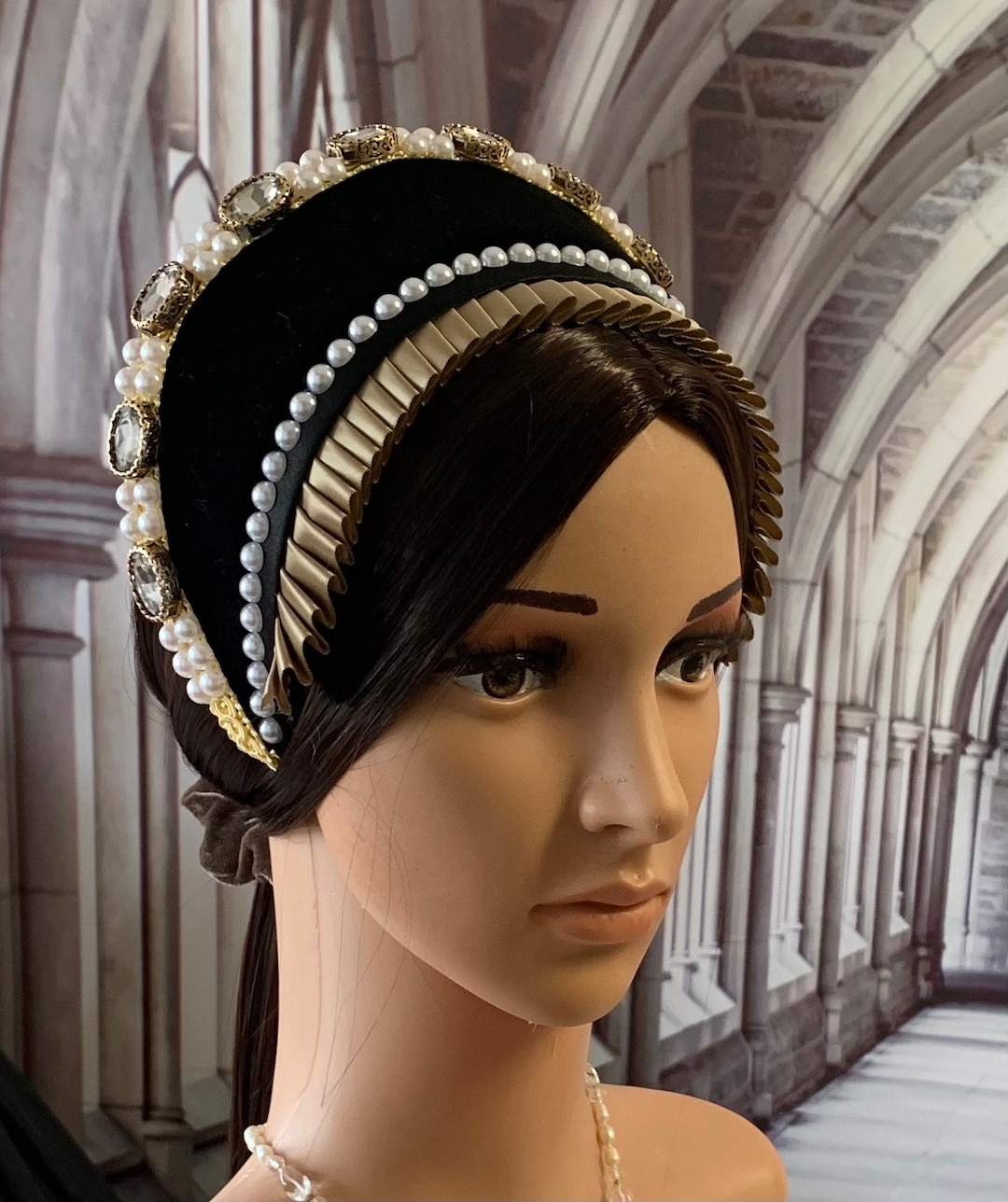This computer-generated image depicts a highly realistic mannequin head, occupying around 75% of the image. The mannequin has a light skin tone, with pink lips and meticulously drawn dark brown eyebrows, complemented by brown eye makeup and long brown lashes. Her striking brown eyes add a layer of realism to her features. She wears a slight pearl necklace around her neckline, adding a touch of elegance.

Her medium to dark brown hair is styled into a formal updo, held by a scrunchie at the back that forms a descending ponytail. The hairdo is adorned with three headbands - the first a simple gold, the second a pearl, and the third a highly ornate combination of gold and pearls. This third headband features a series of repeating patterns: intricate gold circles embedding diamond-like jewels, flanked by sets of two pearls.

The backdrop of the image is an architectural marvel, seemingly an old castle or cathedral with white arches and large, tall windows between each arch. The visible part of the wall is constructed from aged brick, giving a historic ambiance, while the foreground floor is light gray. The combination of the mannequin’s classic elegance and the background’s historic setting implies a period piece, possibly suggesting the mannequin is dressed for a formal occasion from another era.